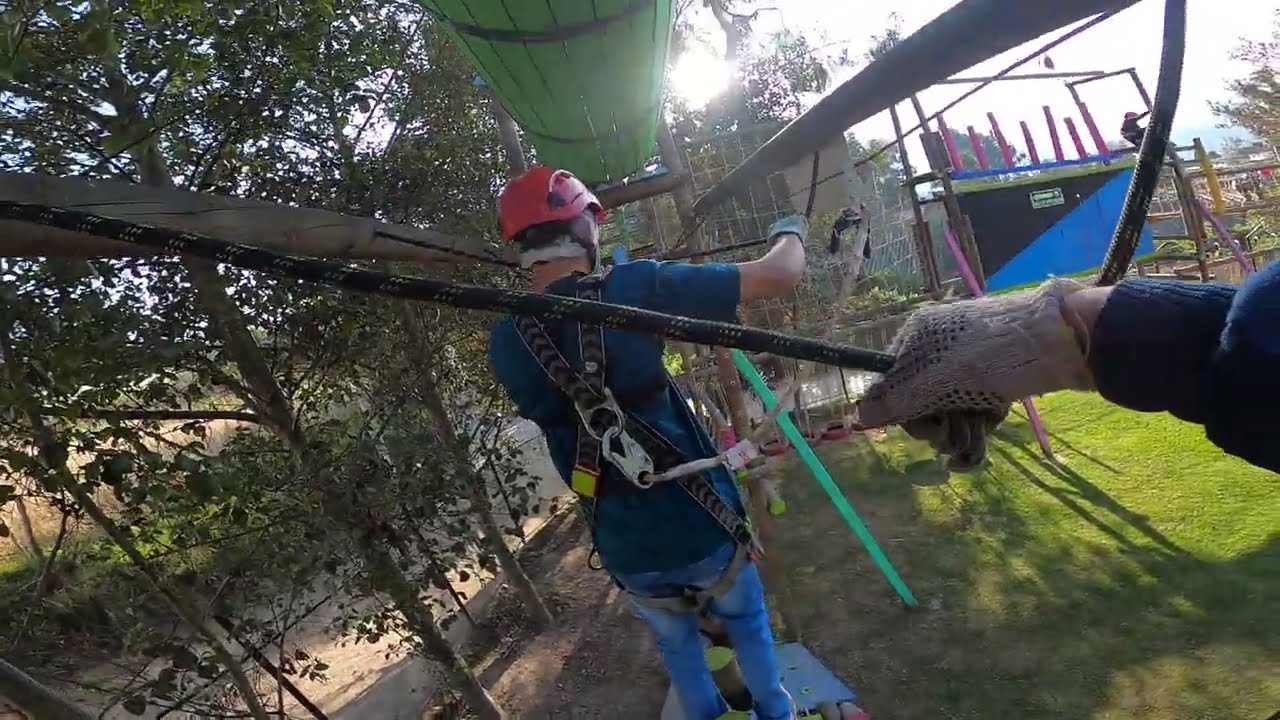This photograph captures an outdoor scene featuring a small-scale ropes and obstacle course. The image is taken from a first-person perspective, evidenced by an arm clad in a blue sweater and knit glove visible on the right, gripping a rope attached to a wooden pole on the left. The scene showcases two individuals navigating the course, both wearing safety harnesses and helmets, with the man ahead dressed in blue jeans, a blue t-shirt, and a red helmet. They are suspended slightly above the ground, maneuvering over what appear to be wooden poles. The course includes various elements such as a climbing net, a wooden tumbler, and a jungle gym-like structure further ahead, suggesting multiple levels of challenges to balance on and climb. The backdrop features landscaped trees on the left and grass covering the ground on the right, indicating a private property or facility, possibly someone's backyard. The bright, midday or early afternoon lighting further emphasizes the vibrant, active setting.